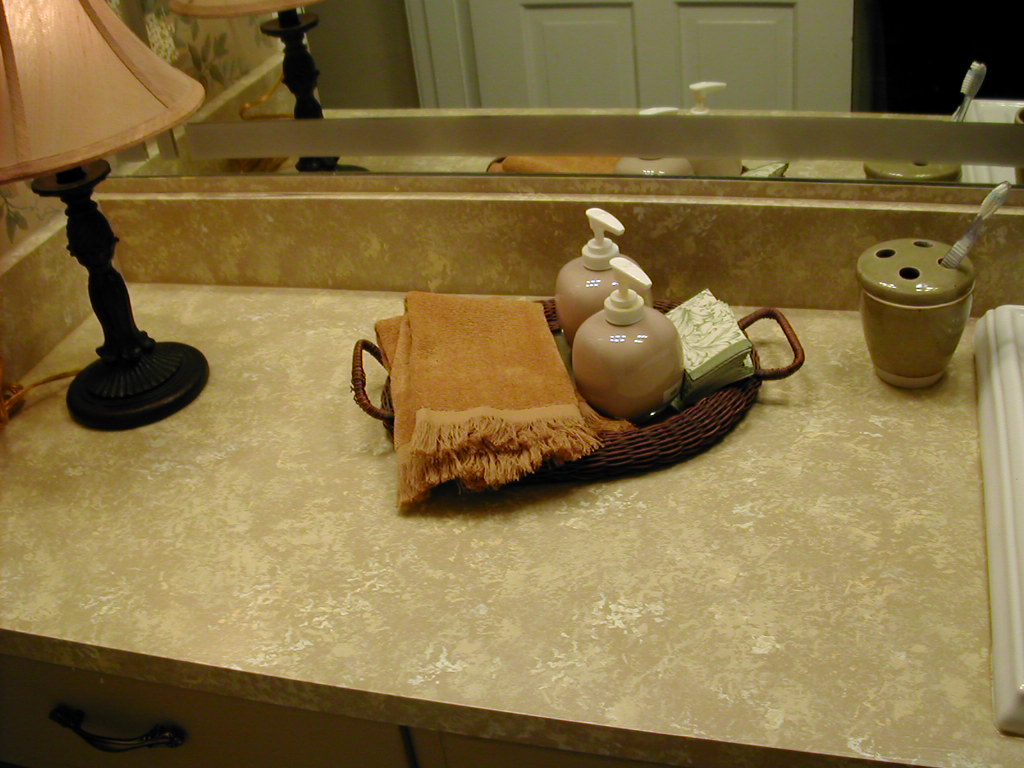The photograph showcases a neatly arranged bathroom countertop, focusing primarily on the cabinet located to the left of the sink. On the extreme right edge of the image, the corner of the sink is visible. Adjacent to the sink sits a small brown cup with four holes in its top, holding a white toothbrush with a clear handle. Moving left, there is a woven basket containing a neatly folded orange towel. Beside the basket are two brown bottles equipped with white pumps, likely containing soap and lotion. A small notepad rests further to the left. The leftmost section of the countertop features a compact lamp with a black base and a tan-colored lampshade, emitting a warm glow. The countertop itself appears to be made of porcelain, decorated with patches of dark gray and white. The background of the scene is dominated by a mirror, reflecting the entire setup and adding depth to the photograph.